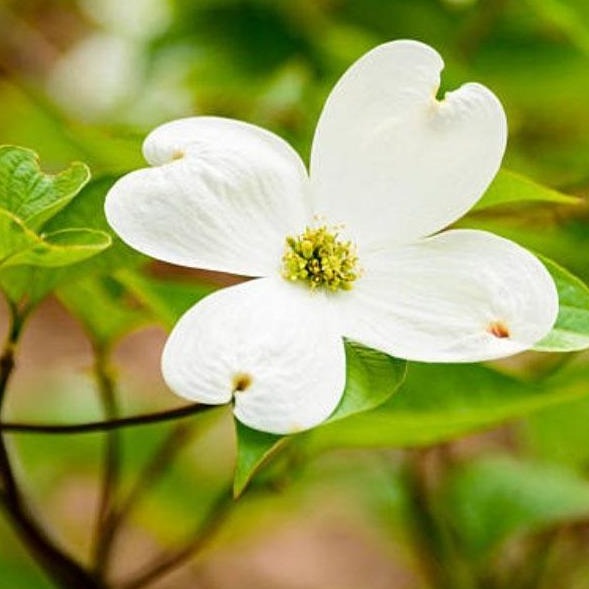This photograph, taken outdoors, features a vibrant close-up of a blooming dogwood flower. The flower's striking white petals, resembling a four-leaf clover, extend in different directions—up, down, left, and right—with each petal having a distinct yellow indentation, forming a subtle cleft. At the center of the flower is a fuzzy yellow-green area, rich with pollen. Surrounding the flower are large, vivid green leaves, some of which are in focus, displaying the fresh hues of spring. Further back, the scene blurs into a mix of greens, browns, and hints of white, suggesting other grasses, plants, and possibly more dogwood flowers of the same kind. The stem of the flower connects to the same plant, emphasizing its natural setting amidst the soft, verdant background. The overall image captures the essence of spring with its bright and lively portrayal of the dogwood bloom.